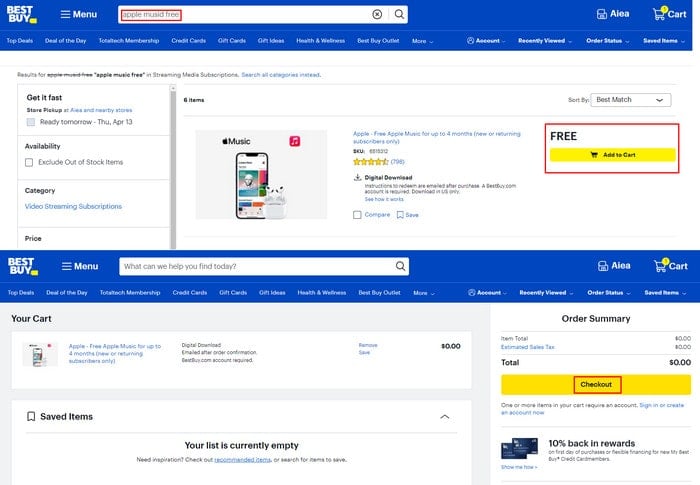In the image, we see a screenshot of an online retailer's website, specifically Best Buy. At the top of the page, there is a distinctive blue bar with the yellow Best Buy logo situated in the upper left corner. The central part of the header features a navigation menu alongside a search bar, where the user has entered the query "Apple Music Free." 

To the right, the user profile name "Aaliyah" is visible, along with a shopping cart icon. The cart appears to contain several items, although the exact number is difficult to determine as it seems to display either '1' or '5.'

Below the header, the search results for "Apple Music Free" are displayed. These results include categories like "Apple Music Free" and "Streaming Media Subscriptions," with prompts to search all categories if needed. The left sidebar offers assorted filters, including "Get It Fast," "Store Pickup," "Area and Nearby Stores," "Ready Tomorrow through April 13th," "Availability," "Exclude Out-of-Stock Items," "Category," "Video Streaming Subscriptions," and "Price."

On the right side of the page, there are specific search results visible. One prominent result is for Apple Music, showcasing an image of an iPhone with headphones alongside the Apple Music logo. The offer advertised is “Apple Music for up to four months free,” available to new or returning subscribers only. This product has a rating of four and a half stars from 795 reviews. A red-highlighted button beneath the description invites users to add the item to their cart for free.

Below this main display, the page transitions into an order summary. It details that the total cost is $0, and includes a brightly highlighted "Checkout" button, inviting the user to complete their order.

In summary, the image captures two consecutive Best Buy web pages: the search results for "Apple Music Free" and the subsequent order summary page showing the free subscription offer ready for checkout.